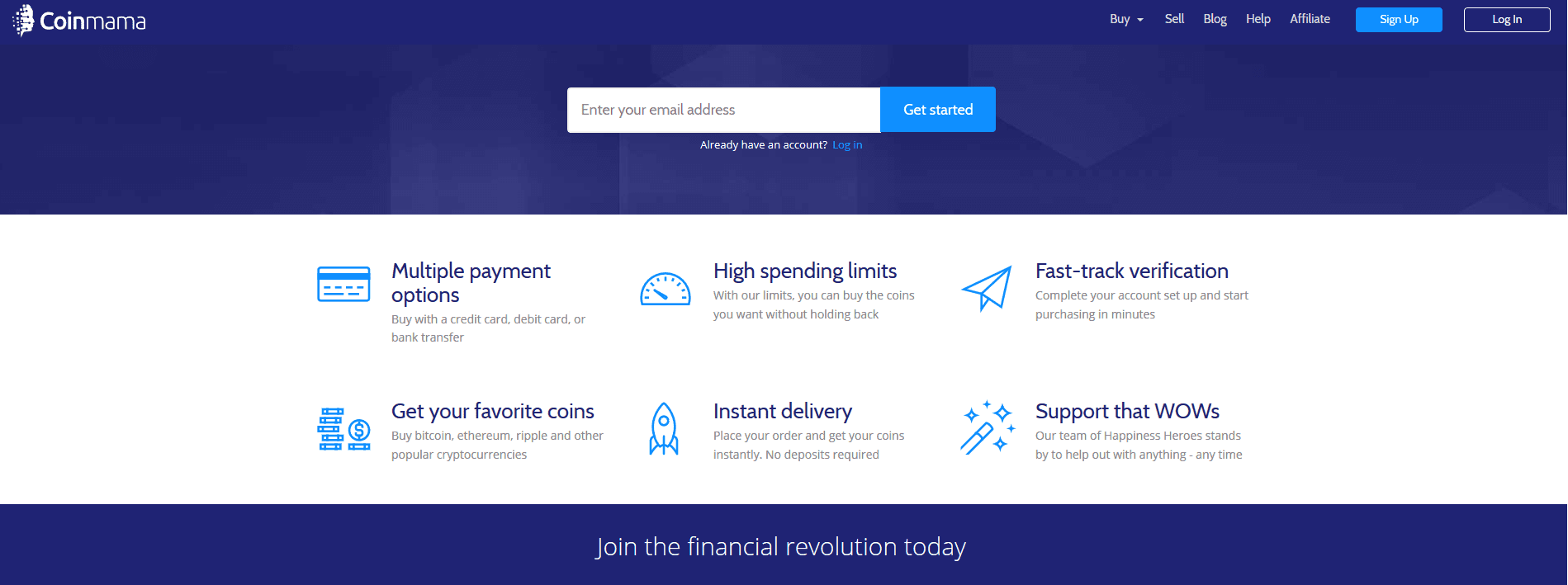The image showcases the top portion of the Coinmama website, predominantly styled in dark blue. The top-most section of the website features a navigation bar occupying about the top 10% of the image. 

- **Top-Left:** The Coinmama logo and name are prominently displayed.
- **Top-Right:** The navigation bar includes links labeled "Buy," "Sell," "Blog," and "Help," with an additional, unreadable link. There are two blue buttons; the lighter blue one says "Sign Up," and the darker blue one says "Log In."

In the top third section below the navigation bar, there is an email subscription form consisting of a text box labeled "Enter your email address" accompanied by a blue "Get Started" button. Below this form, there is a hyperlink stating "Already a member? Log In."

The main content area is structured into a two-row, three-column table listing various features:

1. **Top Row:**
   - Left: "Multiple Payment Options" with a credit card icon.
   - Center: "High Spending Limits" with a tachometer icon.
   - Right: "Fast Track Verification" with a paper airplane icon.

2. **Bottom Row:**
   - Left: "Get Your Favorite Coins" with an icon of coins.
   - Center: "Instant Delivery" with a rocket icon.
   - Right: "Support That Wows" with a magic wand icon.

At the bottom 10% of the image, the dark blue color reappears, displaying a centered white text that reads, "Join the financial revolution today."

This detailed description encapsulates the visual and textual elements presented in the top portion of the Coinmama website as seen in the image.